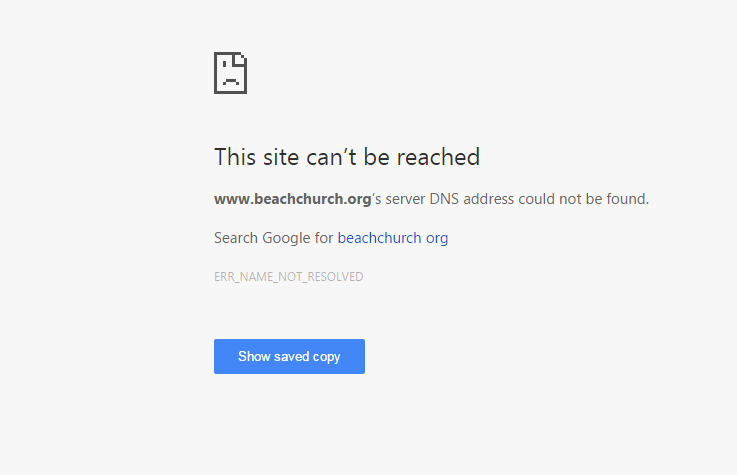The image is a screenshot of a website error message. The background is a light gray, almost off-white color, with a large rectangular or nearly square paper-like element positioned centrally from the left. The paper-like element features a folded-down left corner that resembles an eye, creating the appearance of a right eye and a smiling mouth in the status icon of the page. 

Prominently displayed in bold, larger text is the message "This site can't be reached." Directly beneath this, in darker, bold print, appears the URL "www.beachchurch.org". The message continues in regular font, stating "www.beachchurch.org’s server DNS address could not be found." The text "DNS" is capitalized, emphasizing the technical issue. 

The message then suggests an alternative by stating, "Search Google for beachchurch.org," where "beachchurch.org" is highlighted in blue text, indicating a hyperlink. Underneath, an error code is shown: "ERR_NAME_NOT_RESOLVED," written in all capital letters and underscored.

At the bottom, there is a clickable blue button labeled "Show saved copy" in white text, offering the option to view a previously saved version of the site.